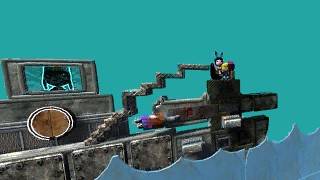In this digitally generated image, we observe what appears to be a scene from a video game or a 3D rendered animation. The background is a turquoise blue, setting a contrasting stage for the foreground elements. At the bottom of the image, there is a 2D cutout resembling ocean waves, depicted in blue with a slightly worn, card-like texture. Central to the scene is a large, dark metal contraption that resembles a steel boat or a piece of machinery with bolts visibly fastened around it. On the deck of this contraption is an oddly shaped staircase leading to a cabin or control area.

Inside this cabin, a character is visible through a window or perhaps a television screen, showing a silhouette with a disproportionately large head. Directly attached to this machinery via what appears to be a crane, there is another platform or chair with a character sitting on it. This character is adorned with a black hat featuring bunny ears and is holding a yellow object. The entire setup has a dark metal gray color, accentuating the industrial and mechanical feel of the scene.